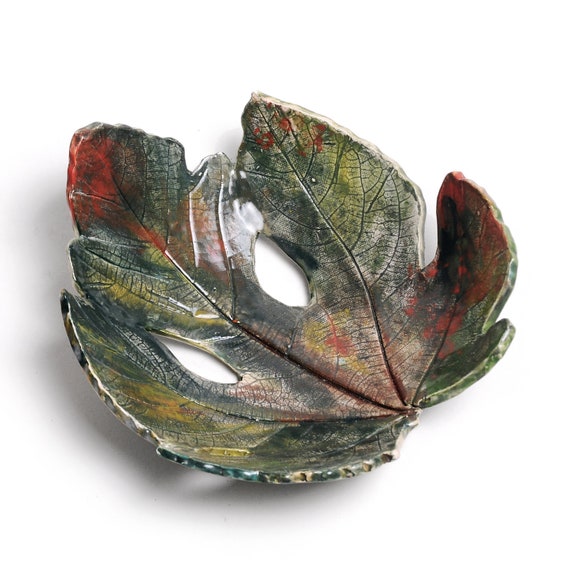This image showcases a small, shallow ceramic dish shaped like an oblong maple leaf displayed against a stark white background. The leaf-inspired dish features curled-up edges, giving it a bowl-like form suitable for holding items that are fairly large, as it has two oval, football-shaped slits cut out in the central area. The leaf's surface is detailed with intricate veins that are dark gray or black, either cut or painted into the ceramic, adding to the realistic depiction of a leaf. The colors on the leaf transition seamlessly from light green to dark green, with accents of reddish orange, yellow, light brown, and sporadic patches of black and white. The leaf's texture is largely glossy due to glazing, although some areas exhibit a matte finish where light does not reflect as intensely. The dish is oriented with the top portion of the leaf situated towards the upper left and the bottom towards the lower right, casting a shadow below and slightly to the left. The overall appearance, blending various autumnal colors and delicate design features, suggests that this may be a decorative piece potentially sold online or featured in a catalog.